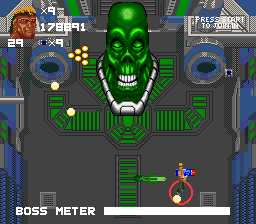The image depicts a vintage video game screen featuring vibrant pixel art. At the center top of the screen, there's a grotesque, glowing green head with eyes closed. The head is distinctly bald with pronounced white teeth, a peculiar triangular nose, and is adorned with a striking silver necklace. The head appears to be emerging from a vast, maze-like area reminiscent of a parking lot, providing open space for movement.

In the bottom-left corner, a character is encircled with a yellow marker, pinpointing their location on the screen. This character has tousled blondish-orange hair and is wielding a futuristic blue gun adorned with a red muzzle. Below this scene, a "Boss Meter" extends almost to its maximum, suggesting an imminent or ongoing boss battle.

The top right of the screen displays "Press Start to Join In," inviting additional players to participate. At the top left, there's an avatar showcasing a man with orange hair, presumed to be the same character controlled by the player. Next to this avatar, the screen displays a score of "178,891" with an adjacent "x9," likely indicating the player's lives or a multiplier. Just left, the number "29" is shown, possibly representing in-game currency, points or another relevant metric.